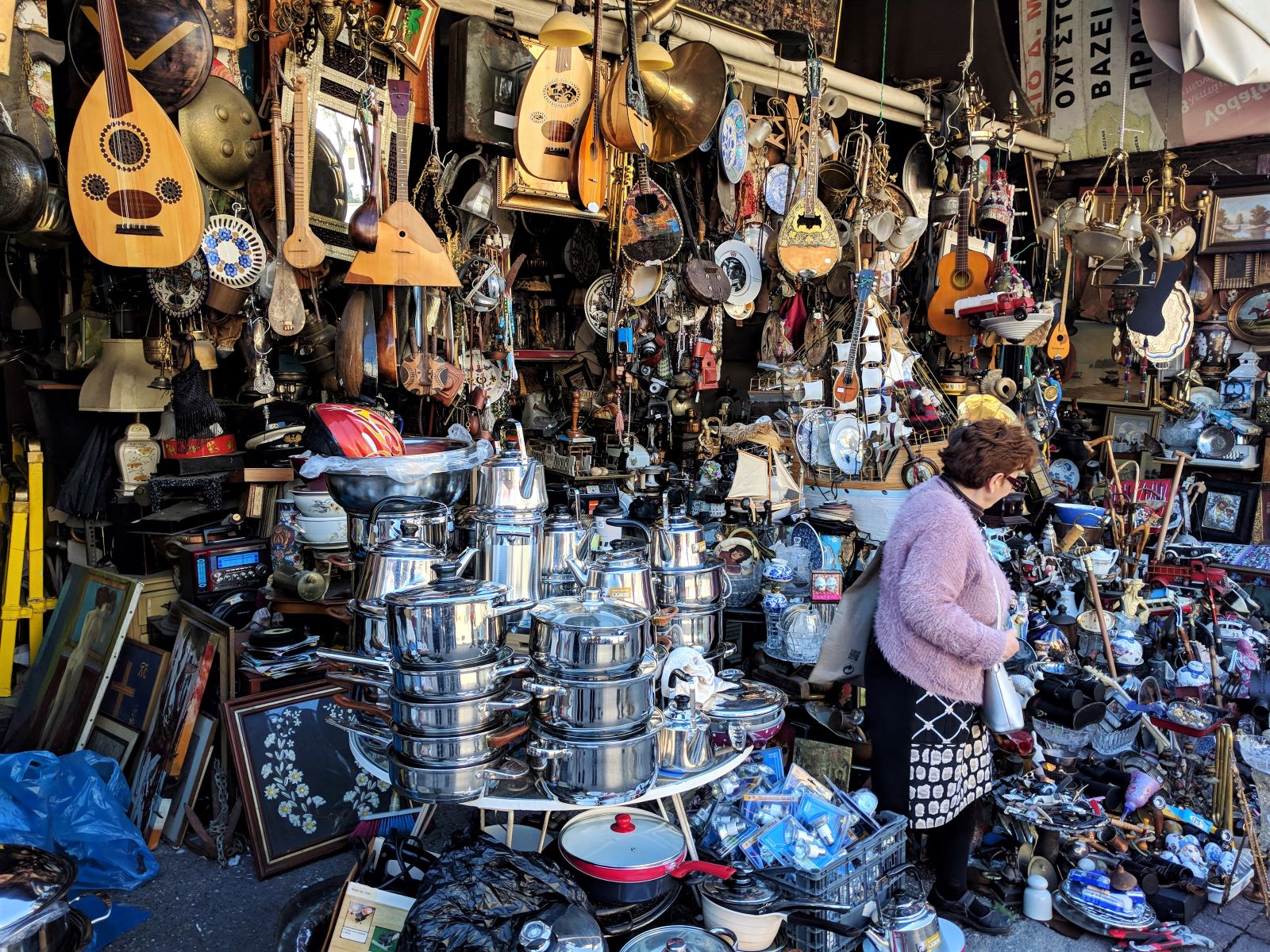The image depicts a bustling, crowded market area, possibly a thrift or antique shop, brimming with an eclectic mix of items. Front and center is an older woman with short, reddish-brown hair, wearing black sunglasses, a fuzzy purple sweater, and a black skirt adorned with white patterns. She carries a white purse over her shoulder. The scene around her is dense with stacks of shiny silver pots and pans, including a notable red frying pan with a clear lid and red handle. Overhead, a myriad of musical instruments – guitars, tambourines, trombones – hang amid various lamps and chandeliers. On the left side of the image, numerous framed pictures are visible, adding to the impression of a seemingly endless collection of random, intriguing objects. The overall atmosphere is one of cluttered charm, with every inch of space utilized, leaving little room to navigate.